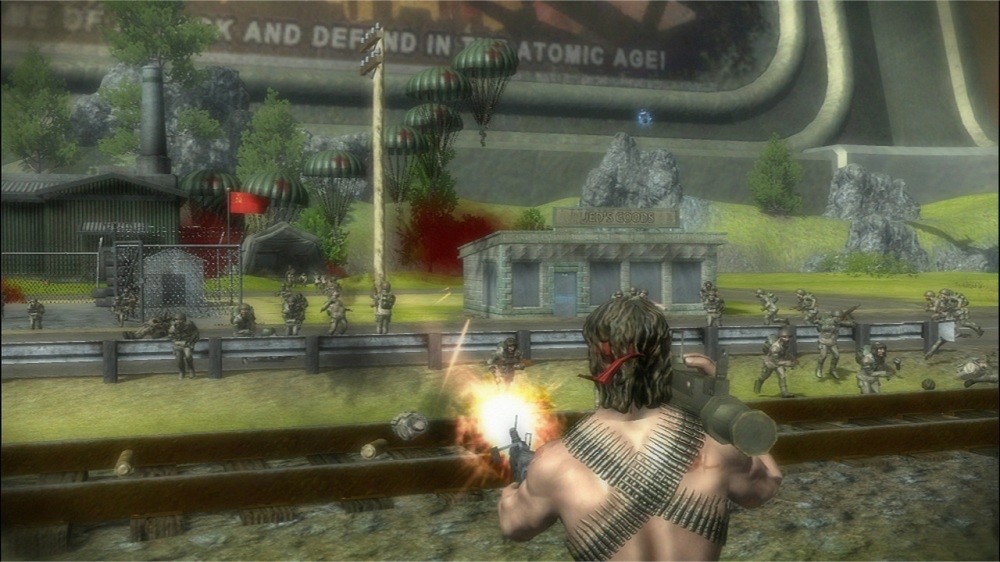The image is a detailed screenshot from a video game set in a war or attack scenario. The main character, a muscular man with shoulder-length brown hair and a red bandana tied around his head, stands with his back facing the viewer in the center bottom area. He is shirtless, revealing several rounds of ammunition strapped across his chest in an X pattern, extending around his back. In his left hand, he is seen firing a gun with visible flames, while a bazooka rests on his right shoulder. The background reveals a chaotic battlefield with several soldiers dressed in green, some equipped with helmets, advancing towards the main character. The setting includes various buildings, a smokestack, green grass, and a fenced area, along with a set of brown railroad tracks laid over rocks. Text in the image reads "Defend in the Atomic Age," further emphasizing the wartime atmosphere.